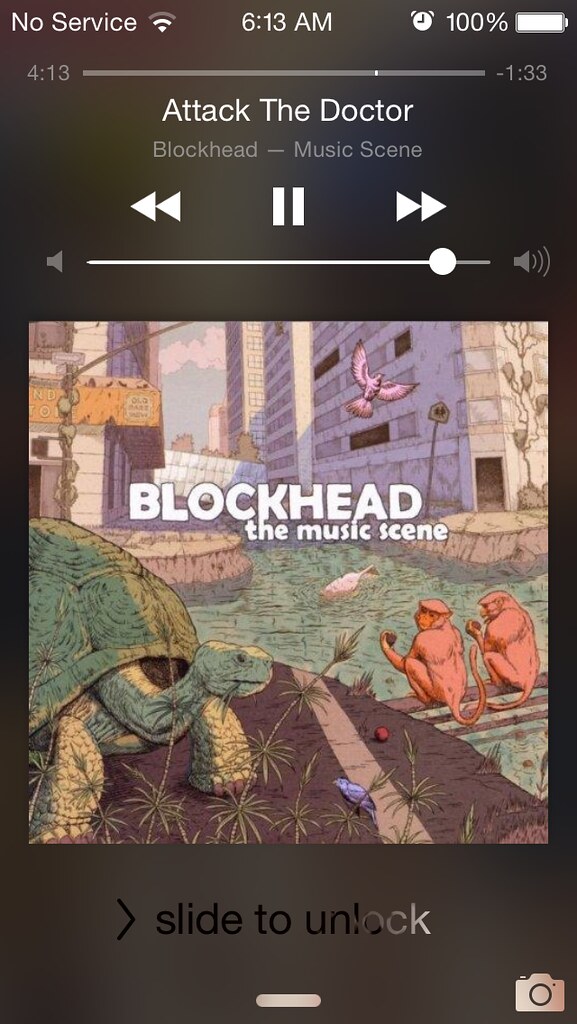The image shows a smartphone screen with no service at 6:13 AM and a fully charged battery at 100%. The screen displays music controls with "Attack the Doctor" and "Blockhead - The Music Scene" indicated. In the center, album cover art is prominently featured, showcasing a turtle eating grass, two orange monkeys, a purple bird flying, and a city scene taken over by nature with vines and grass climbing up buildings. The setting is likely indoors, hinted by the detailed phone display. The main colors in the album artwork include black, orange, green, pink, blue, and brown. At the bottom of the screen, it says "slide to unlock."